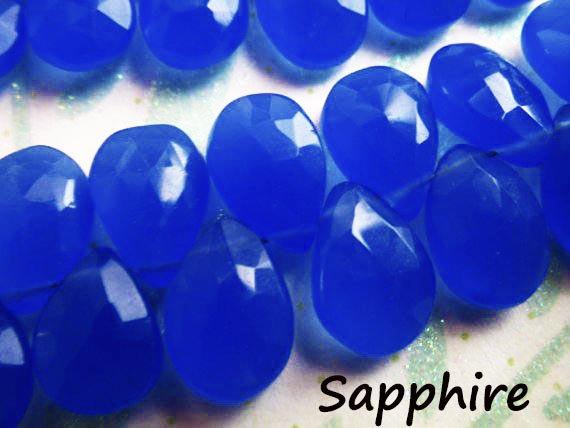This image features an up-close view of radiant blue teardrop-shaped sapphire gemstones. The sapphires are arranged in two staggered rows that run across the center of the photo, creating a striking visual of nested point-up and point-down gems. The background is a glittery surface with a light mint green and white cream color, adding a sparkling contrast to the vivid blue of the sapphires. Light reflections highlight the smooth, faceted surfaces of the gems, creating a shiny, almost reflective appearance. In the bottom right-hand corner of the image, the word "sapphire" is displayed prominently in black font, confirming the identity of these gemstones. The overall setting suggests a jewelry display, possibly akin to what one might find in a jewelry store.